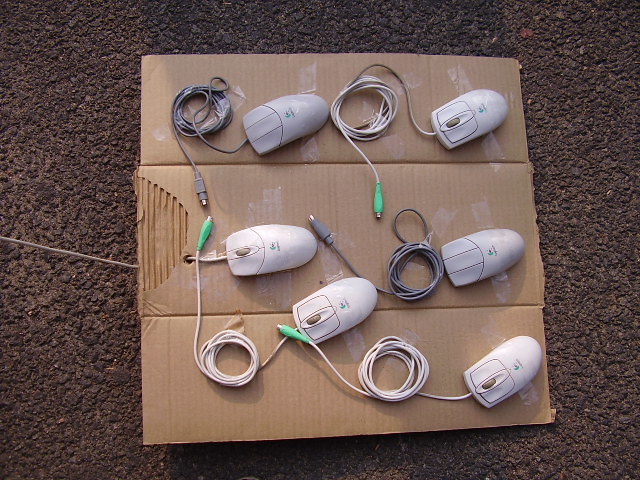The image presents a top-down view of six vintage computer mice affixed to a flap of rough cardboard, which is placed on dark brown tarmac. The cardboard is loosely divided into three sections, with two mice per section, and shows signs of wear, including a tear and missing pieces on the left side. Each mouse is either white or gray, with four featuring scroll wheels and two without. They are secured to the cardboard with clear tape, both at the mice and on their coiled cords. The cords—some white, some gray—terminate in green ports, indicative of old PS/2 connectors from the late 90s to early 2000s. Everything in the image, from the taped mice to the textured concrete background, is captured in meticulous detail, yet devoid of any explanatory text or additional imagery.